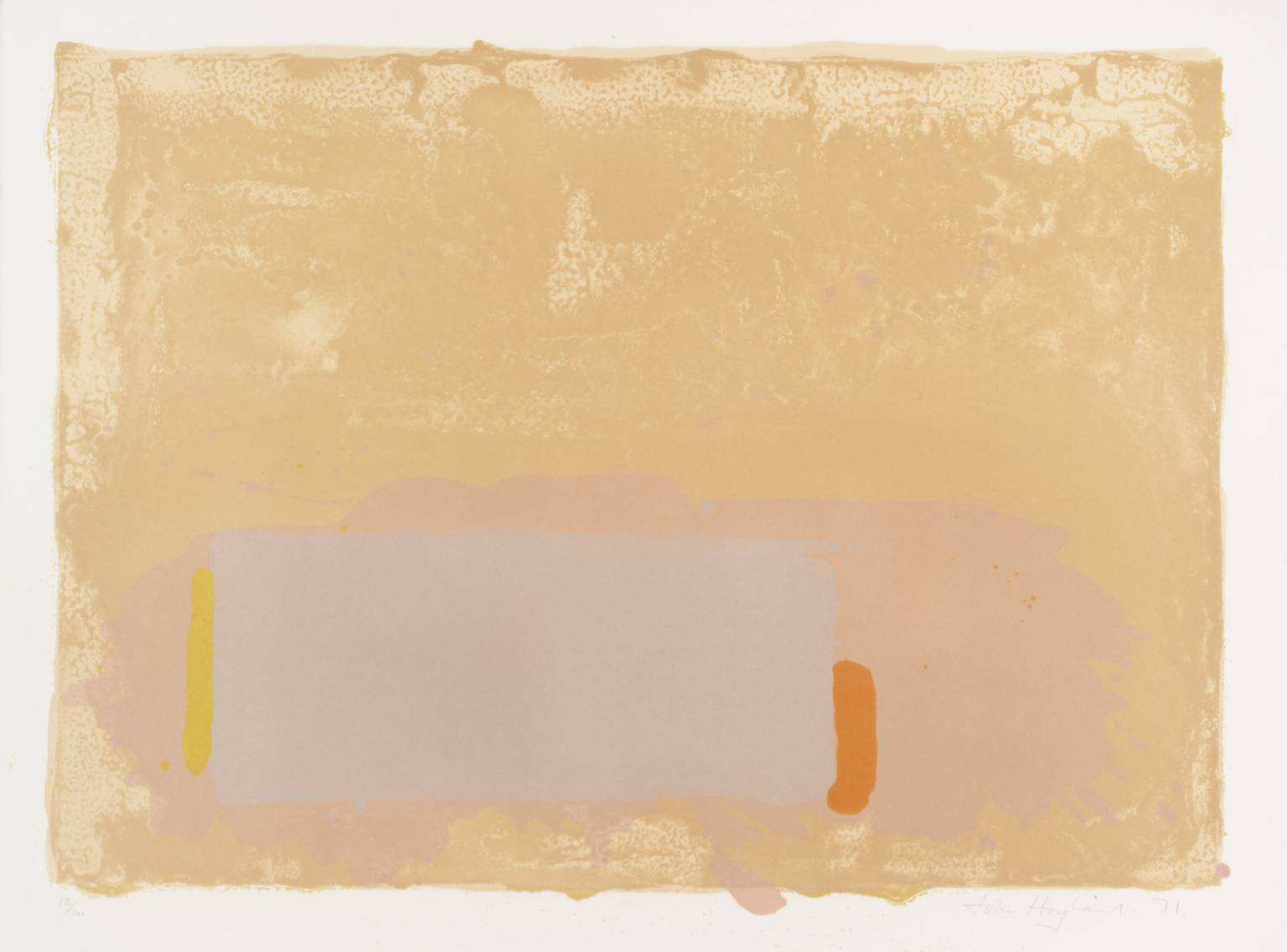This abstract painting features a central beige rectangle set within a light gray backdrop with a white border. The beige rectangle appears to be applied haphazardly, creating a sense of spontaneity. In the lower left corner of the beige rectangle, there is a light gray square. Overlapping this area, a narrow vertical yellow band borders the left side of the gray square, while an orange or rust-colored line borders the lower right side of the gray square. Additionally, a blob of lighter gray appears behind the gray square, adding a splotchy and irregular texture to the composition. The overall effect is a layered, textured piece with an emphasis on soft, blended colors and shapes without clear, hard-defined lines.